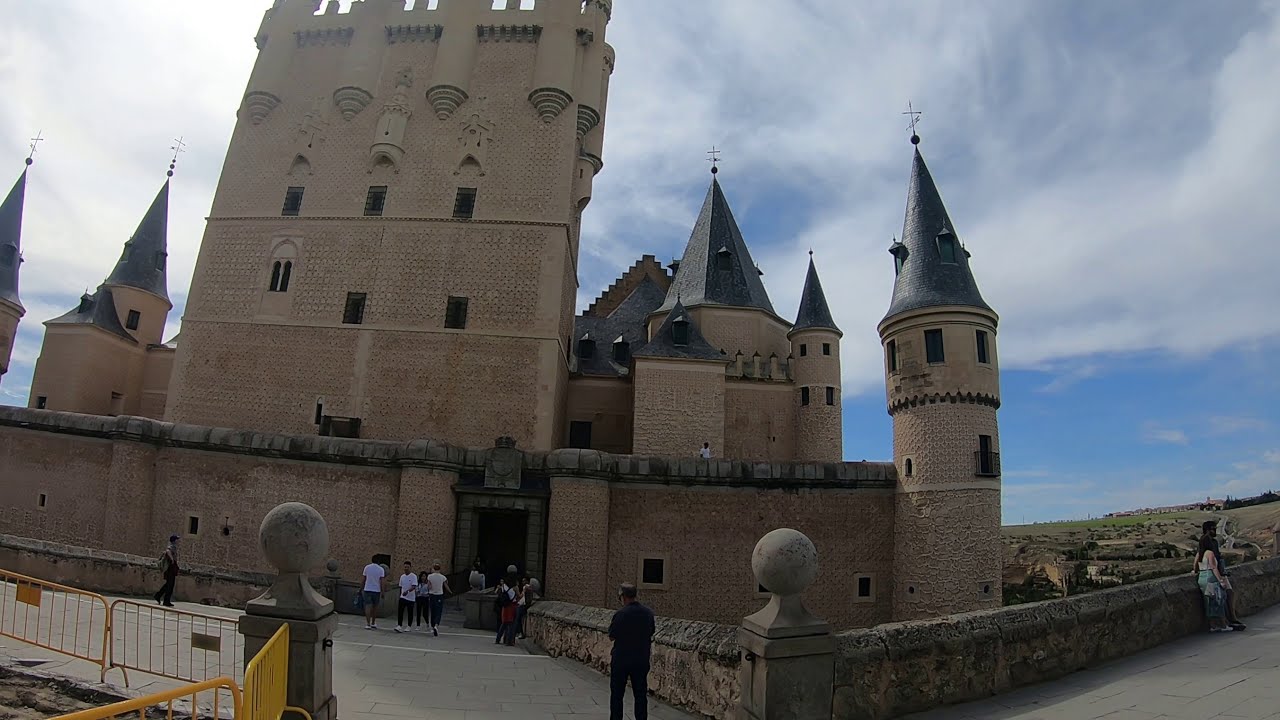The image captures a large, classical European castle, possibly located in Germany or Spain, characterized by its imposing beige brick or stone facade adorned with bluish domed, cylindrical ceilings and pointed spires topped with crosses. The castle, a likely medieval structure, features a multi-layered design including tall outer walls and rectangular windows. Tourists can be seen entering through a prominent front gate in the central portion of the compound, which is surrounded by other spires and parapets. A large green meadow expands in the background under a sunny sky dotted with wispy clouds. People, casually dressed in t-shirts, wander around and lean on a stone fence. Temporary yellow metal fencing on the left side, typically used for crowd control, and a dark-clothed man with his back to the camera in the foreground add to the bustling scene of visitors exploring the historic site.